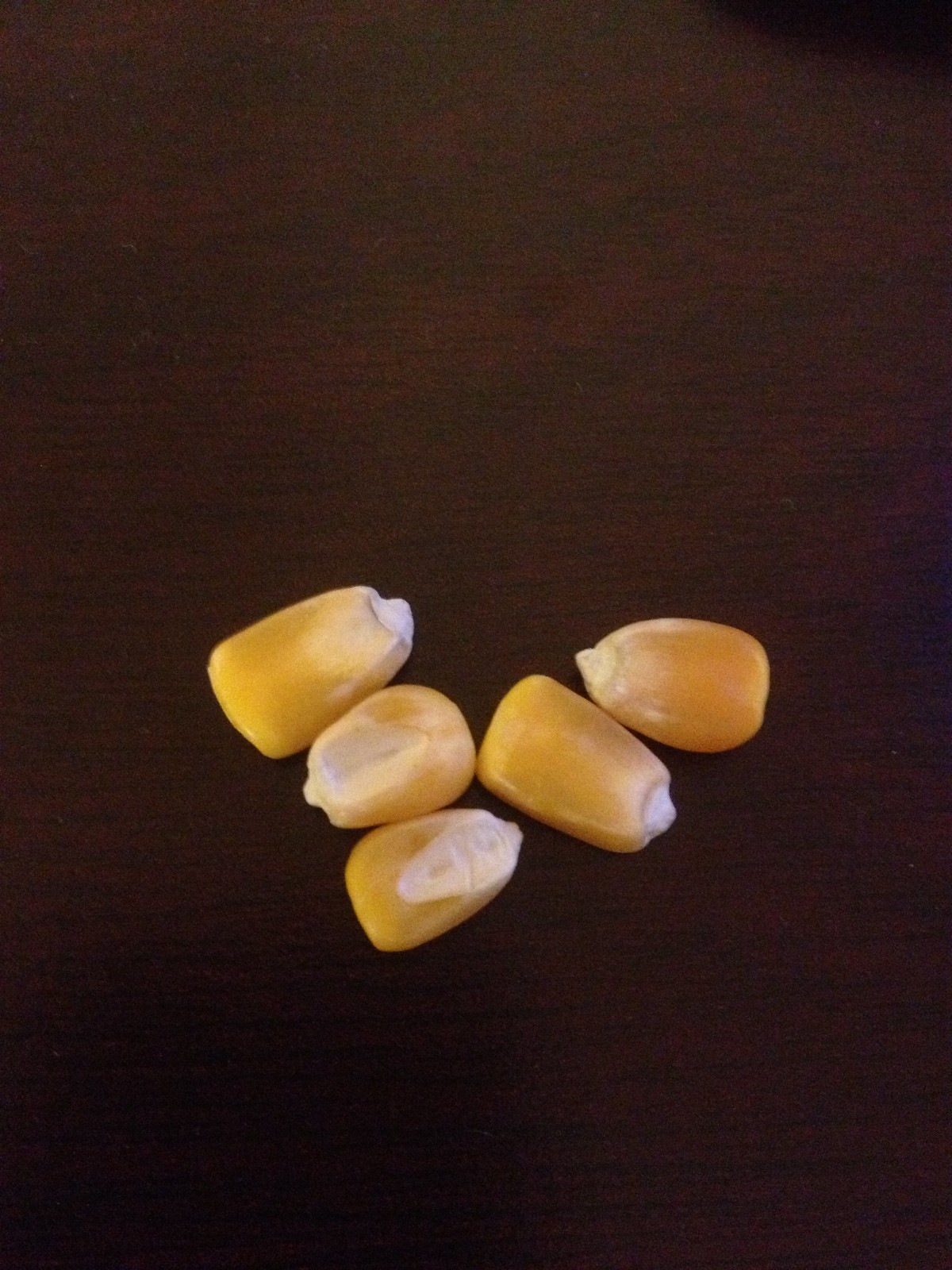This slightly blurry, vertically oriented snapshot features five dried, unpopped corn kernels arranged in a V shape on a dark brown wooden table, possibly cherry wood or mahogany with prominent black wood grains. The kernels vary in color, transitioning from a darker yellow at the base to lighter yellow and ending with white tips. They are grouped such that three kernels form the left diagonal side of the V and two form the right diagonal side, all touching, with alternating directions. Notably, two of the kernels appear to have a broken piece coming off them, adding a subtle texture to the image.